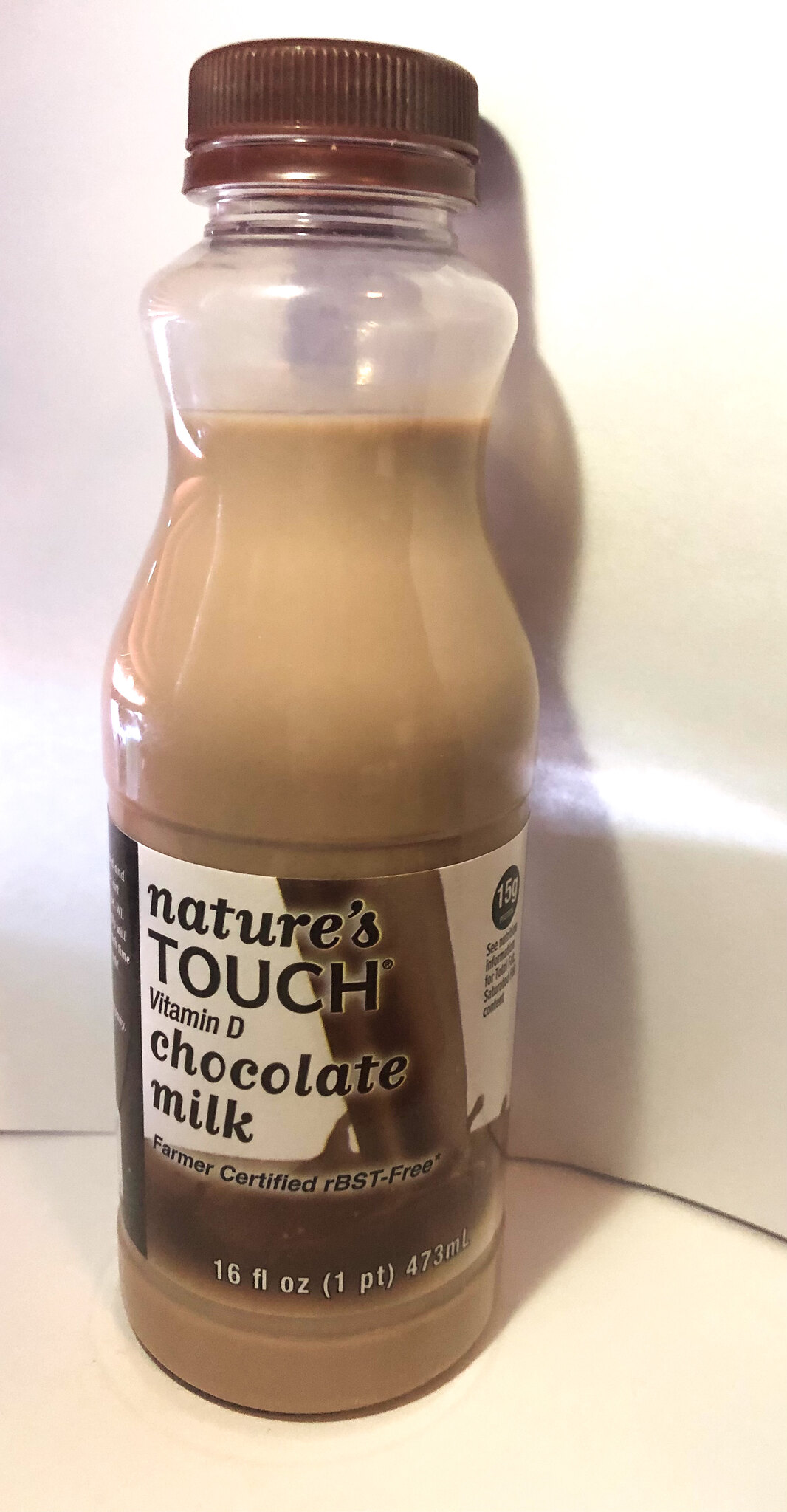This image features a zoomed-in view of a 16-fluid ounce (473 ml) bottle of Nature's Touch Vitamin D Chocolate Milk. The bottle, made of clear plastic, reveals the light brown chocolate milk inside. It has a dark brown screw-on cap with an intact seal, though it appears a small amount of the milk has been consumed. The label, situated towards the bottom of the bottle, clearly states "Nature's Touch Vitamin D Chocolate Milk," "Farmer Certified RBST-Free," and the volume measurements in fluid ounces, pints, and milliliters. The bottle is positioned against a white background that seems to blend into a countertop or ledge, with varying shades of white and yellowish light reflecting off the surface. Additionally, the label mentions 15 grams of something, though this detail is partially obscured. The composition and lighting of the photo highlight the bottle and its contents, making it the focal point.